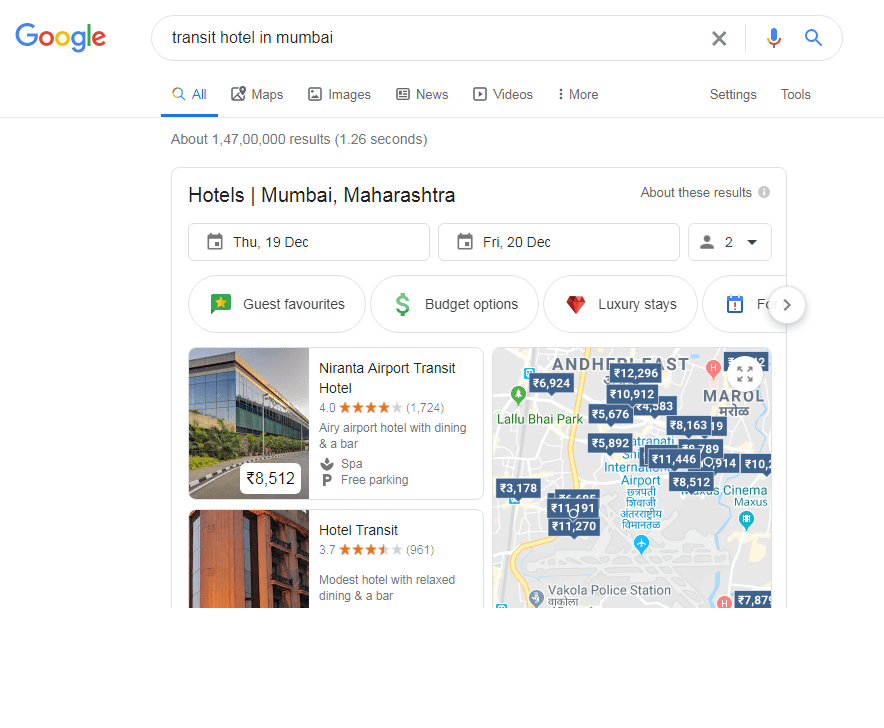Screenshot of a Google search result for "transit hotel Mumbai":

At the top, the search bar reads "transit hotel Mumbai" with the Google logo on the left. To the right of the search bar, there's an 'X' icon for clearing the search and a microphone icon for voice input. The search category is set to "All."

Below, the search results indicate 1,047,000 results found in 1.26 seconds. The first visible result is for "Hotels Mumbai Maharashtra," displaying the check-in date as Thursday, December 19th, and the check-out date as Friday, December 20th. It also shows a drop-down menu for selecting the number of people, currently set to two.

A prominent green oval-shaped badge labeled "Guest Favorites" with a yellow star icon sits below the date selection. Next to it, there are buttons for navigating "Budget Options" and "Luxury Stays," and a right arrow button for further options.

The top two hotel listings are displayed under "Guest Favorites." The first one is the "Niranta Airport Transit Hotel," which features a modern building with glass windows facing a road. The hotel has a rating of 4.0 out of 5 and advertises amenities like spas and free parking. The price shown is ₹8,512.

The second listing is for "Hotel Transit," rated 3.7 out of 5. This hotel is described as having modest accommodations with relaxed dining options.

A map to the right shows various hotel locations in the Mumbai area, with prices marked for easy comparison.